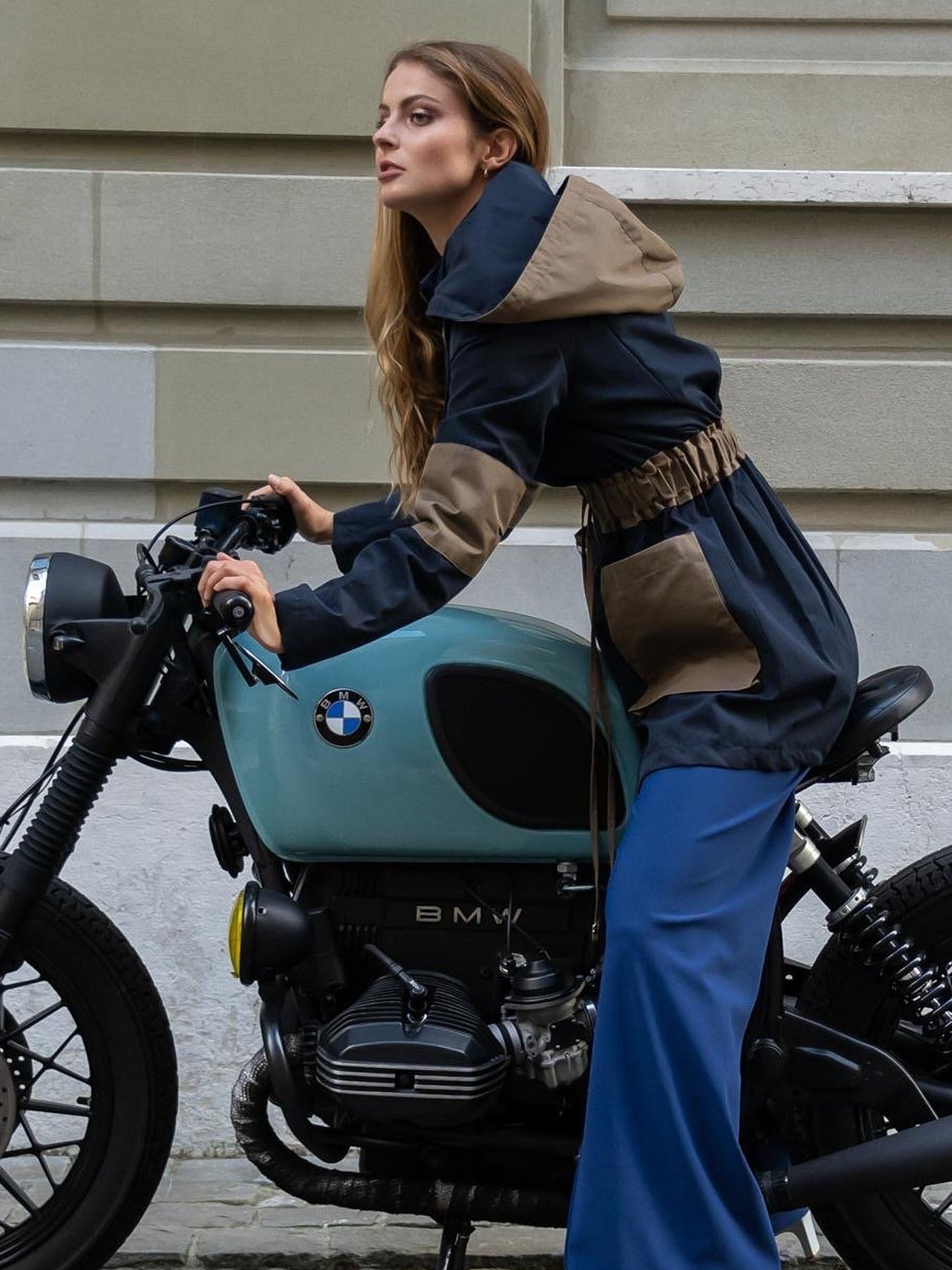This color photograph captures a young, slim woman with long, flowing light brown hair and a pretty face, posing atop a BMW motorcycle, suggesting a fashion shoot. The motorcycle, featuring a distinctive teal-colored fuel tank adorned with the iconic silver BMW logo and blue-and-white checkered emblem, also showcases low handlebars, a vintage single headlight, and black tires with black spokes. The woman is dressed in stylish flowy, wide-leg blue linen pants and a dark navy blue parka-style jacket, detailed with tan elbow patches, a brown hood, brown pockets, and a brown waistband. She sits on the black leather seat of the bike, with the kickstand down and her feet touching the ground, adding to the poised aesthetic of the scene. The backdrop includes a greenish-sided concrete or stone building with a white stone retaining wall beside a cobblestone street, enhancing the picturesque, vintage feel of the composition.